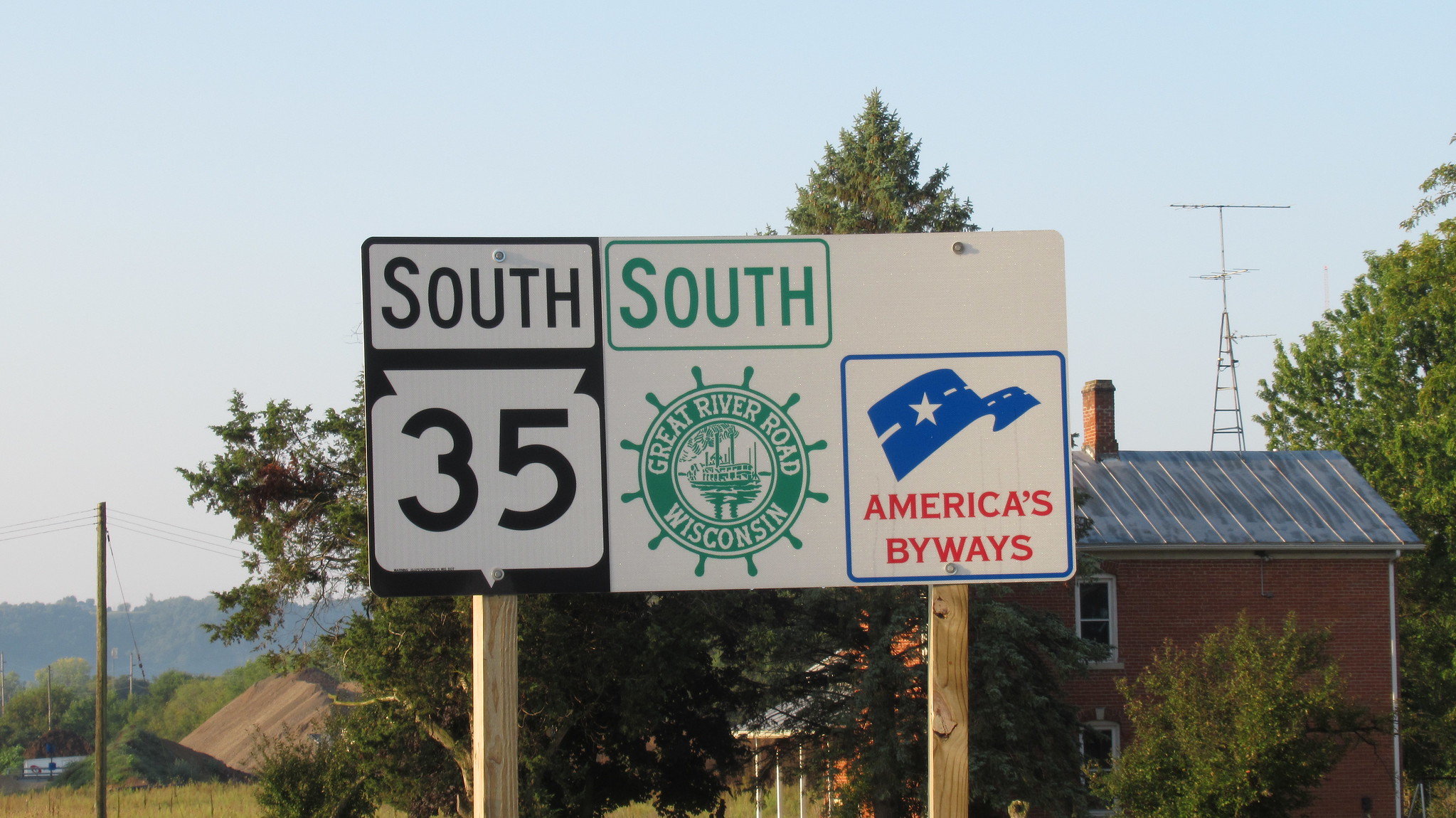A detailed photograph captures a rural scene that appears to be from the United States. Central to the image are several road signs with distinct markings. Behind these signs, there is a red brick house characterized by its tin roof and brick chimney. Also visible is a radio tower rising behind the house, adding to the quaint rural atmosphere. To the left side of the photograph, there is a utility pole strung with power lines. The road signs stand out with their contrasting designs: one has a white background with black lettering, indicating "South 35." Another sign features green writing and reads "South Great River Road, Wisconsin." Adjacent to it, a distinct sign bordered in blue displays a stylized blue road with a star replacing the usual white lines. This sign bears the red inscription "America's Byways." The combination of these elements paints a vivid portrait of a serene yet junction-centric locale in rural America.